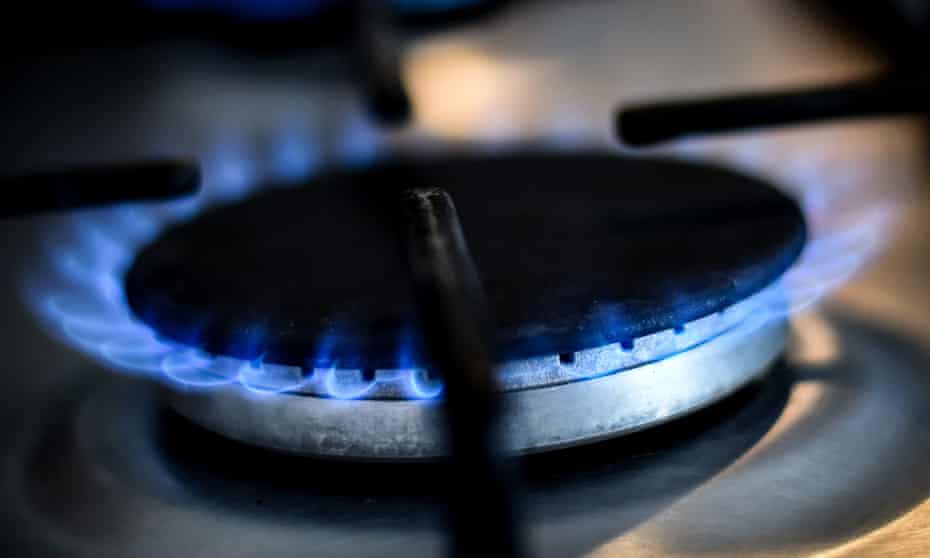The image showcases a close-up photograph of a lit gas burner on a stovetop. The burner, which is square-shaped and made of stainless steel, features a central round metal burner. Blue flames are visible, emanating from various small black holes around the perimeter of the burner. Despite the image being blurry and out of focus, making it difficult to discern finer details, one can see that the burner supports a black disc on top. Radiating from the burner are black metallic arms that form the stovetop grate, designed to hold a pot or pan over the flame. The stovetop itself appears to be a typical metallic surface, further emphasizing the functionality of the gas burner setup.